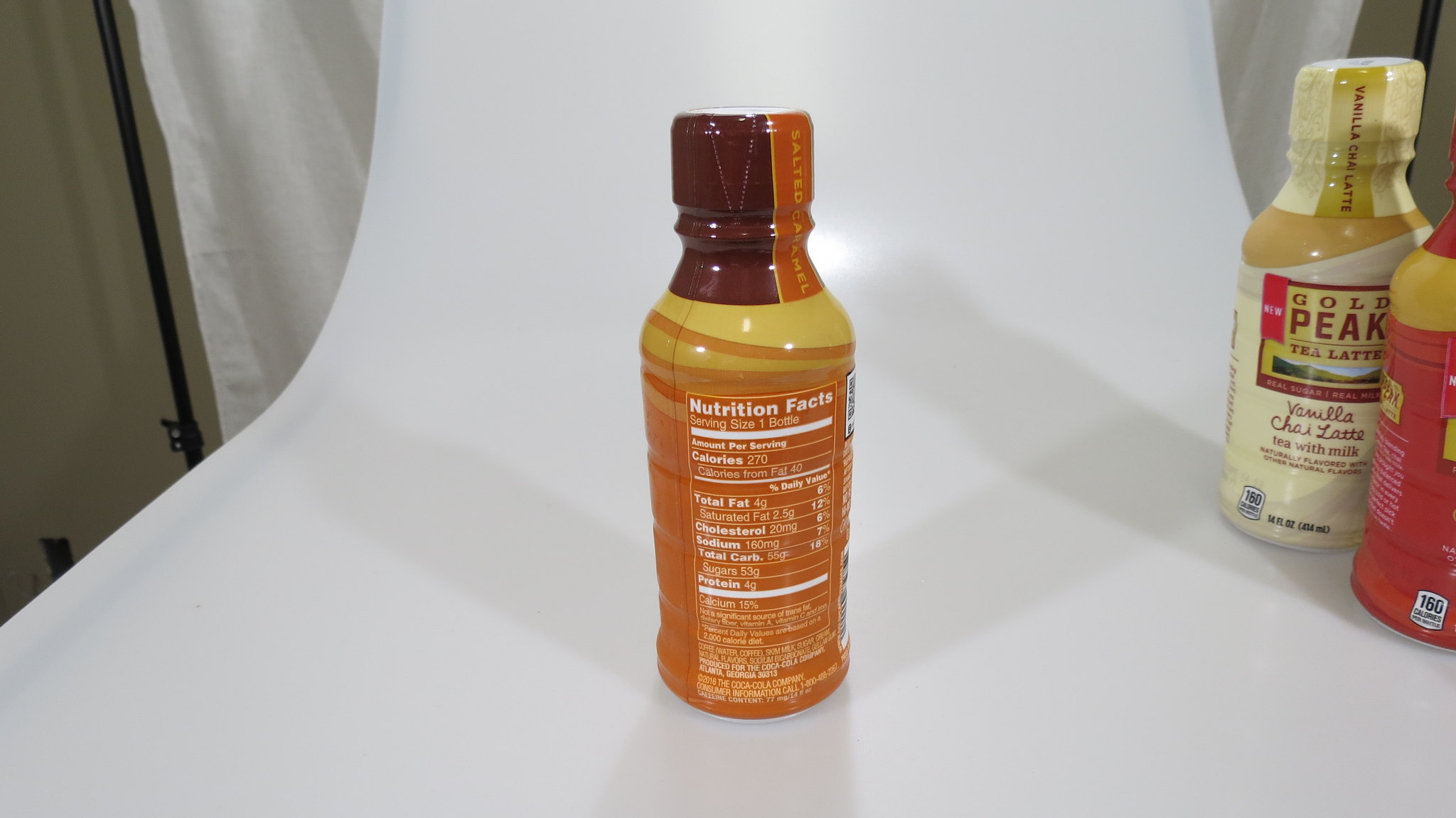In this meticulously staged photo, an individual is engaged in capturing product images, specifically focusing on a bottle of tea. The featured bottle displays its Nutrition Facts label prominently on its back, ensuring all crucial information is visible. It is set against a pure white photodrop background, intended to create a seamless, transparent effect once photographed. The bottle itself is a vibrant fusion of yellow and orange, crowned with a brown plastic wrap encasing the cap. At the top of the bottle, a vertical rectangular orange label brandishes the flavor, "Salted Caramel," in bold lettering. Adjacent to the primary bottle, on the right side of the composition, rests a Gold Peak Tea Latte bottle, identified as a Vanilla Chai Latte by its label. Alongside it is another striking bottle, distinct in hues of red and yellow, adding an additional splash of color to the otherwise minimalist setup. The overall arrangement is designed to be visually appealing and informative, ensuring each product is represented with clarity and detail.